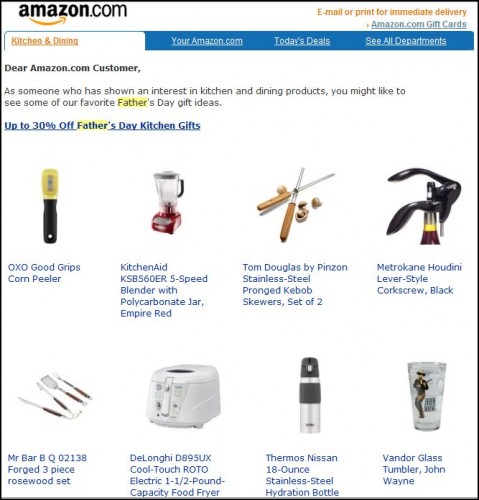This is a detailed photographic depiction of a webpage from amazon.com. At the top of the page, we see the iconic Amazon logo, presented in black, lowercase font with the well-known yellow arrow underneath. To the right of the logo is a yellow text prompt stating, "Email or print for immediate delivery." Below, there's a blue hyperlink that reads "Amazon.com gift cards.”

The header of the page features several tabs, with "Kitchen and Dining" highlighted in yellow. To the right of these tabs, a blue banner displays "Your Amazon.com." The page includes a section, "Today's Deals," located within a category labeled "Departments."

The main content begins with a greeting, "Dear Amazon.com Customer." It follows with a personalized suggestion for those interested in kitchen and dining products, promoting their "Favorite Father's Day Gift Ideas," as part of a limited-time sale offering up to 30% off on select kitchen gifts. This link is emphasized with a hyperlink.

The page showcases a selection of recommended items for Father's Day, enumerated as follows:
- An "OXO Good Grips Corn Peeler,"
- A "KitchenAid Five-Speed Blender with Polycarbonate Jar in Empire Red,"
- A "Tom Douglas by Pinzon Stainless Steel Prolonged Kebab Skewers, Set of 2,"
- And a "Houdini Lever Style Corkscrew in Black."

The layout effectively communicates targeted promotional content, aiding users in finding suitable gifts for Father's Day within the kitchen and dining category.